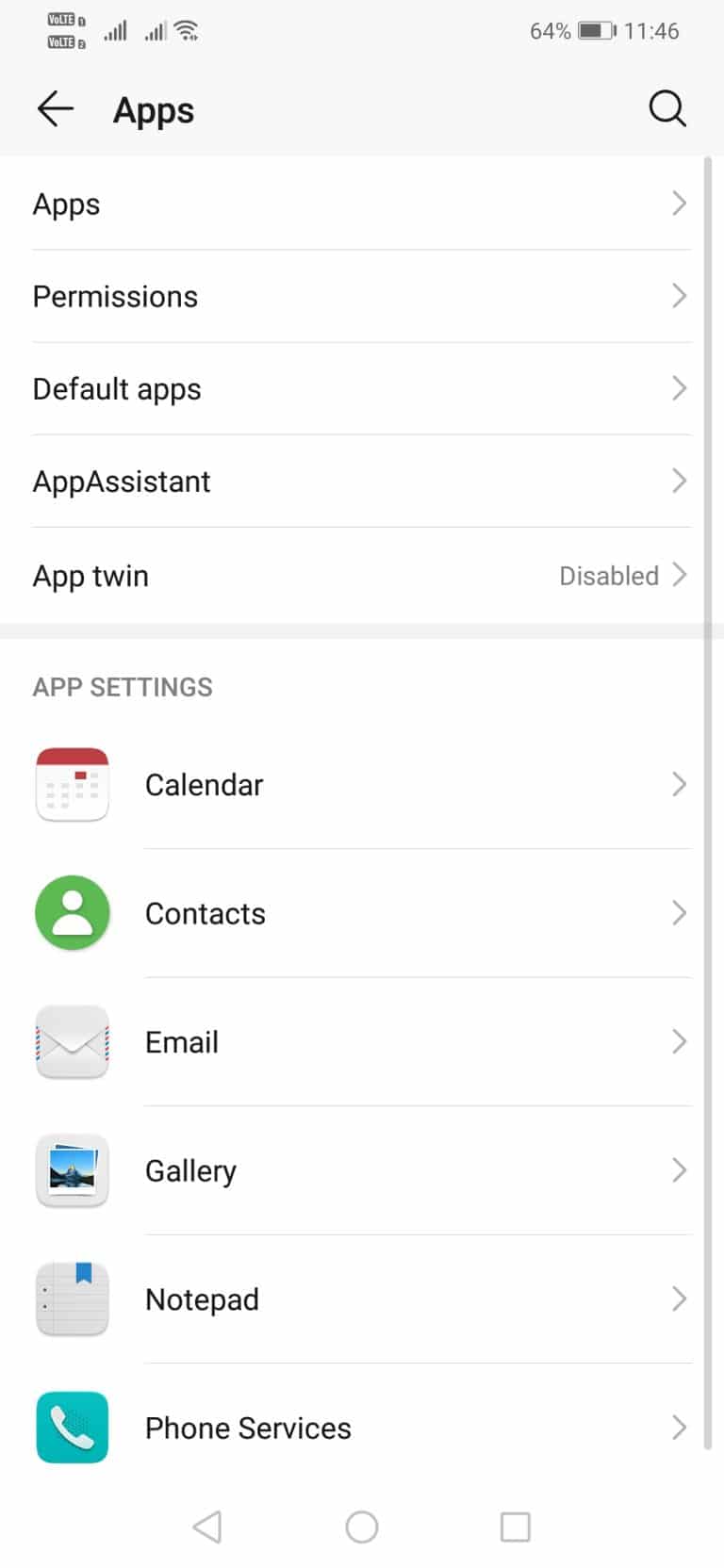This screenshot from a cell phone displays an 'Apps' menu interface. The top section, labeled 'Apps' in black font with a capital 'A,' features a back arrow to the left of the word 'Apps.' Below this header is a sequential list comprising various app-related settings:

1. **Apps** 
2. **Permissions**
3. **Default Apps**
4. **App Assistant** (written as one word)
5. **App Twin** (with an adjacent space indicating it is disabled, accompanied by a right-pointing arrow)

Each item in this list has a right-pointing arrow, suggesting that additional options or settings can be accessed by selecting them.

Further down, another section titled 'App Settings' features a range of specific applications, each accompanied by a right-pointing arrow for further configuration:
- **Calendar**
- **Contacts**
- **Email**
- **Gallery**
- **Notepad**
- **Phone Services**

These arrows indicate that additional settings or options can be explored for each listed application.